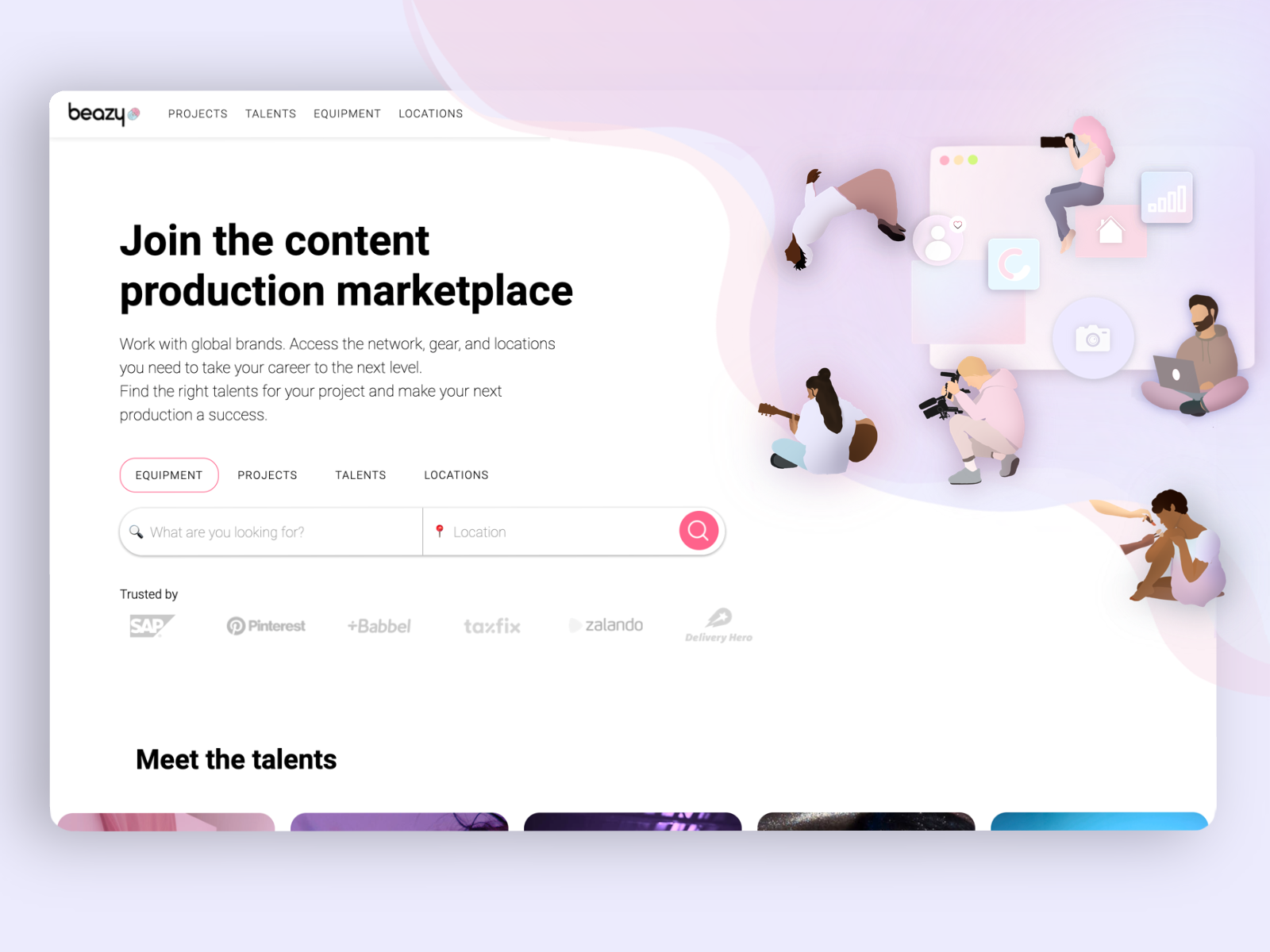The screenshot depicts a website called "Busy Be Easy." The primary content is hosted on a white panel adorned with a pink swirl design that cascades down from the upper left corner, reminiscent of dripping paint. The website showcases various categories such as Projects, Talents, Equipment, and Locations.

Prominently displayed are graphics depicting individuals engaged in diverse activities: performing a backflip, taking a photograph, working on a laptop, recording a video, and playing the guitar. Additionally, the interface features several icons, including a home button graphic and a graph icon.

A text section reads, "Join the Content Production Marketplace. Work with global brands. Access the network, gear, and locations you need to take your career to the next level. Find the right talents for your project to make your next production a success." 

The navigation highlights four main options: Equipment (encased in a pink capsule), Projects, Talents, and Locations. There is also a distinctive search feature, represented by a round button with a magnifying glass icon and a pink search bubble for location queries.

Notably, the website lists its trusted partners, including prominent names like SAP, Pinterest, Babbel, Topics, Alando, and one other that is not fully legible.

Towards the bottom of the screenshot, you see a section titled "Meet the Talents," featuring five colored photo squares, partially cut off at the bottom. This design appears intentional as more pink design elements are visible below, indicating that scrolling might reveal the rest of the images.